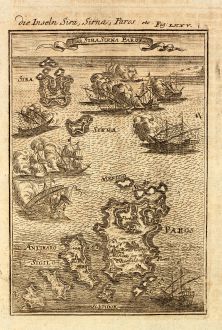This image is a vertically rectangular print reminiscent of a page from an old book, set on aged light brown paper with darker brown smudges that accentuate its age. The print is bordered first by a brown edge and then a black line, creating a dual-layered frame. At the very top, an archaic-looking italic font, possibly in Dutch or German, displays text that's difficult to decipher due to its faintness and intricate cursive style. Below this header, there's a banner with additional text that's equally challenging to read. 

Occupying the majority of the print is a detailed engraving of an ancient map. The map features a cluster of islands towards the bottom, with the intricate details of their shorelines outlined in black. Scattered across the map are various depictions of old sailing ships, some of which appear to be floating, while others look like they might be wrecked, giving a sense of the perilous waters they navigate. The overall impression is one of an antiquated, simple map that, despite its small and faded presentation, strikes a nostalgic chord with its depictions of maritime exploration.